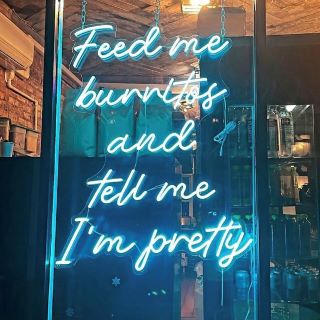The image depicts a neon sign hanging outside a restaurant, viewed through glass windows bordered in brown wood. The sign, illuminated in light blue with white accents, reads from top to bottom: "Feed me burritos and tell me I'm pretty." The sign is suspended by three chains, visible in the photograph as they hang down from above. Inside the restaurant, to the right, there is a cabinet with glass shelves, displaying several rows of what appear to be either liquor bottles or cans. Directly in the background, there are three white bags that look like coffee bags, partially obscured by the neon sign. To the left, an air conditioning unit is mounted at the top, with a white pipe extending towards the back of the building. Wooden planks make up the ceiling, and a yellow light shines down, enhancing the retro ambiance of the space. The overall scene through the windows gives a glimpse into a cozy, eclectic interior marked by a mix of modern and vintage elements.